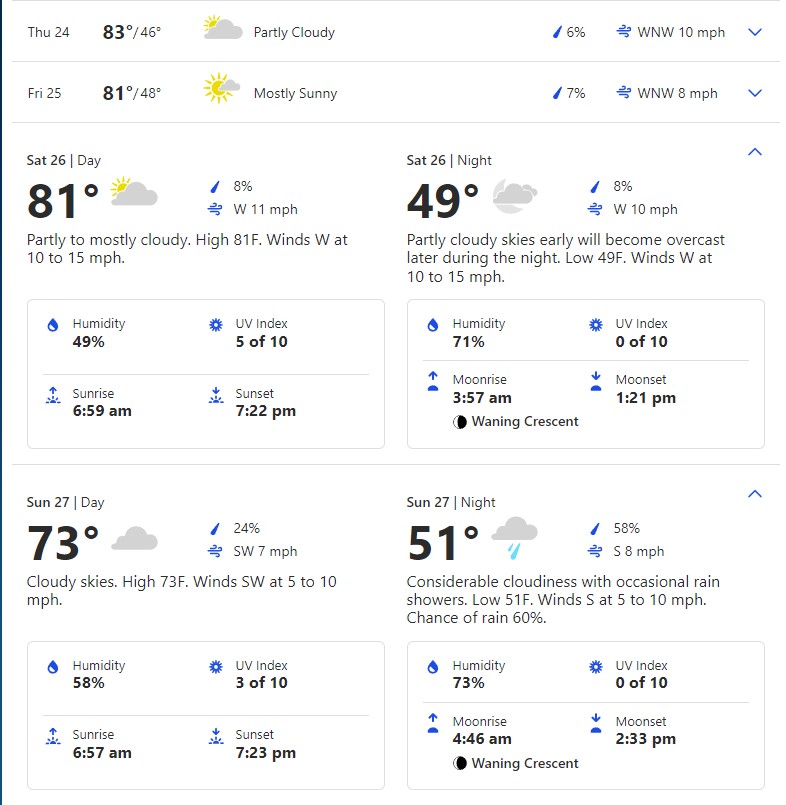This image depicts a detailed weather forecast page, providing comprehensive information for multiple days. For Thursday, the 24th, it shows a high temperature of 83°F and a low of 46°F with a partly cloudy emoji. There is a 6% chance of rain, indicated by a raindrop icon, with winds coming from the northwest at 10 mph. A drop-down arrow is present, likely for accessing detailed hourly forecasts.

For Friday, the 25th, a similar layout is seen with temperature, cloudiness, chance of rain, and wind information. 

The forecast for Saturday, the 26th, stands out with an expanded section, revealing more detailed information. It describes the weather as partly to mostly cloudy with a high of 81°F and winds from the west at 10 to 15 mph, providing a range for wind speeds.

Below the daily forecasts, there are additional boxes displaying humidity percentage, UV index, and precise times for sunrise and sunset. This detailed information is provided for both Saturday and Sunday, including both high and low temperatures.

The text is primarily in black on a white background, with additional data such as humidity, moonrise, moonset, and UV index highlighted in blue. This detailed presentation ensures that users have all the necessary weather information, including the potential intensity of UV rays and exact timings for sunrise and sunset.